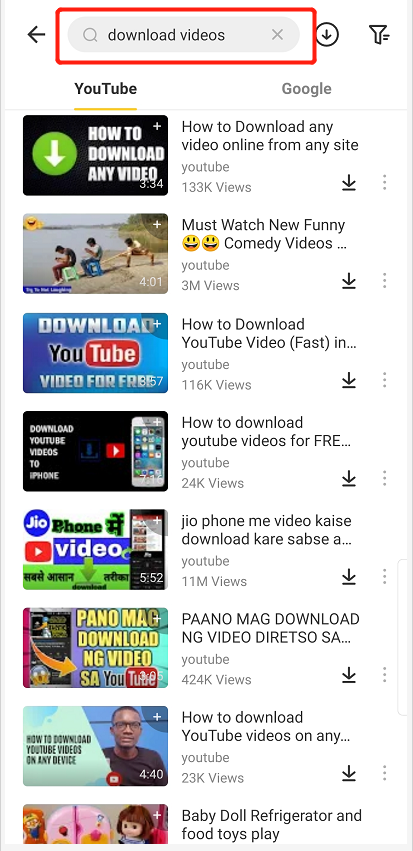A screenshot of a smartphone display showcasing a video download search interface. At the top of the screen, there is an elongated, oval-shaped search bar containing the text "download videos," flanked by a grayed-out magnifying glass icon on the left and an equally grayed-out Xbox logo on the right. This search bar is outlined in a conspicuous red rectangle to draw attention to it.

To the immediate right of the red box, an arrow points left, accompanied by a circular icon with a downward-pointing arrow. Further right is a small funnel icon, oriented downwards, indicating a filter option. Directly beneath these elements, there's text; "YouTube" appears on the left, highlighted in black to show it is selected, while "Google" on the right is grayed out, indicating it is not selected.

Below this section, there is a prominent black box containing the title "How to Download Any Video." Adjacent to the left of this text is a green circle with a white downward-pointing arrow inside. To the right, it reads "how to download any video online from any site." Underneath, it displays "YouTube, 133k views." Following this, a downward-pointing arrow with a line beneath it, and three small vertically-aligned dots are visible, indicating menu options.

Further down, there's another image of people seated by a beach. To its right, the text reads "Most Watched New Funny Comedy Videos" with two smiley faces, followed by more video listings extending to the bottom of the screen. The partial final video preview shows the top part of a toy doll with the accompanying title to the right: "David Dollar Refrigerator and Food, Toys, Play."

This detailed description captures the elements and layout of the phone screenshot, emphasizing the interface's visual and functional components for video downloading and browsing.